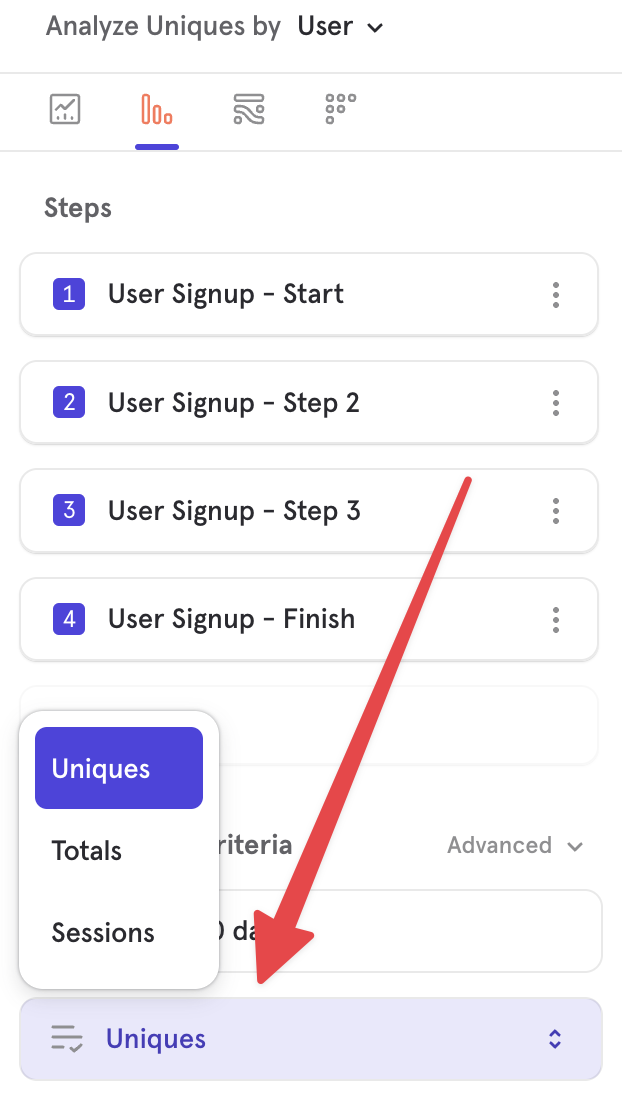This image is a screenshot of the Google Analytics app interface, specifically focusing on user analysis. At the top of the interface, the title "Analyze Uniques By" is prominently displayed, with an adjacent drop-down menu currently set to "User." Below, a highlighted bar graph icon, denoted by a blue underline and a red highlight, indicates that the graphical view is active.

On the left side, the text "Steps" is presented in large, bold letters. Beneath it, four vertically arranged and numbered boxes represent the different stages of the user sign-up process. Each box is bordered in blue and includes a number, starting with "1: User Sign Up - Start," moving to "2: User Sign Up Step 2," followed by "3: User Sign Up Step 3," and finally, "4: User Sign Up - Finish." Each stage box also displays a menu icon on the far right.

Towards the bottom of the screenshot, a bar labeled "Uniques" is highlighted in purple, accompanied by a clicked menu option on the left. This action has revealed a pop-up box above it, showing three selectable metrics: "Uniques," "Totals," and "Sessions," with "Uniques" currently selected. To the right, a prominent red arrow, edited onto the image, points directly at the "Uniques" option, drawing attention to this specific metric.